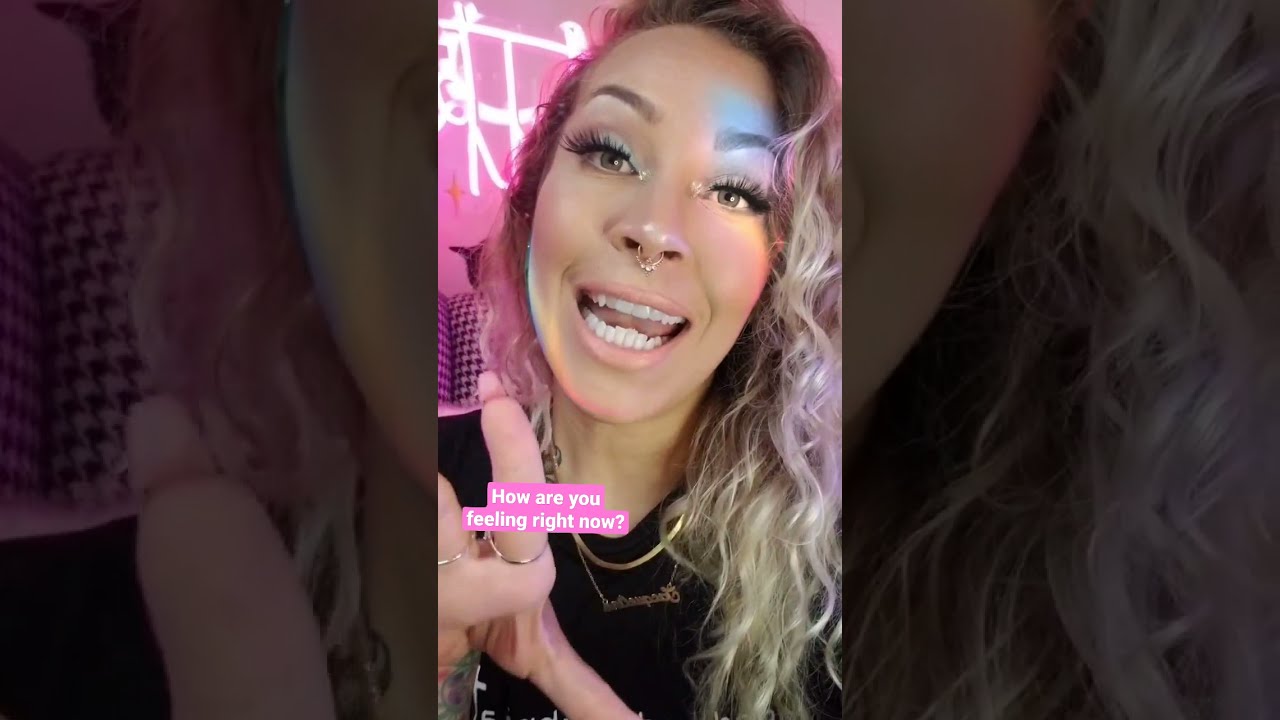This still from a TikTok video features a close-up, portrait-oriented shot of a young woman, likely in her 20s or 30s, with long, wavy blonde hair that cascades past her shoulders. Her hair has hints of pink hues, especially noticeable on the right side. The woman has light brown skin and wears makeup, including pink lipstick. She also has a nose ring piercing between her nostrils and gold necklaces around her neck. Her attire includes a black t-shirt.

In the image, she is mid-sentence with her mouth open and teeth visible, and she is holding up her right hand, fingers forward, as if emphasizing a point. Several rings adorn her fingers. The background features an artistic, pink-colored backdrop with white, non-English characters or scribbles. Overlaying the image is a pink text box in the bottom-left corner with white text that reads, "How are you feeling right now?" The borders on either side of the central image are darker, zoomed-in fragments of the woman's face, contributing to a layered, photoshopped aesthetic.